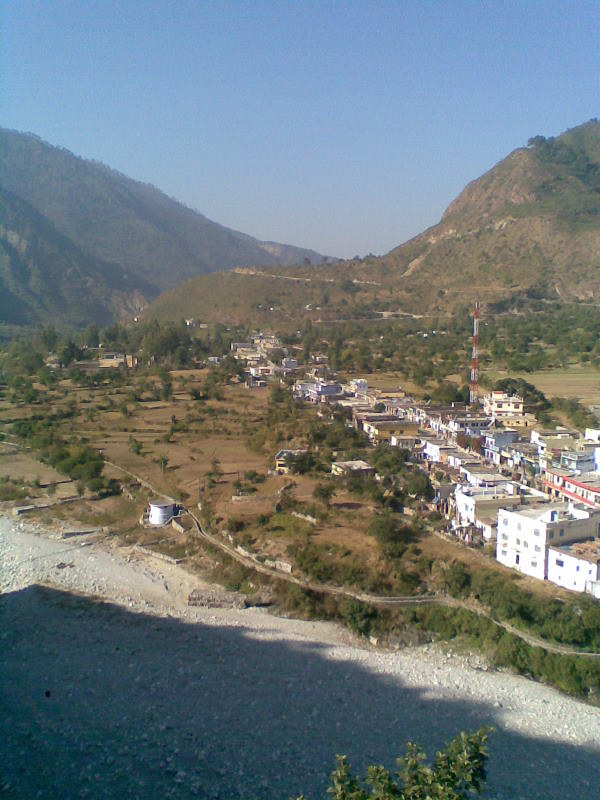The photograph portrays a scenic, high-altitude view of a desert town nestled in a valley, framed by towering greenish hills and shadowed mountains under a cloudless blue sky. The sky occupies the top third of the image and fades to a light gray-white near the horizon. Below, there's a shadowed, rocky expanse with small pebbles, leading to a vibrant green area filled with shrubs, pine trees, and scattered larger trees, particularly on ridgelines. A single, long dirt road cuts through this lush vegetation and connects to a strip of old-style square buildings typical of a historic mining town, stretching centrally through the town parallel to the road. Further back, the green hills give way to more vegetation and open flatlands, dotted intermittently with foliage. In the foreground, closer to the photographer, a serene blue river with a rocky coast completes the picturesque landscape. The distant mountains rise on both sides of the photograph, creating a natural frame that enhances the depth and beauty of the scene.